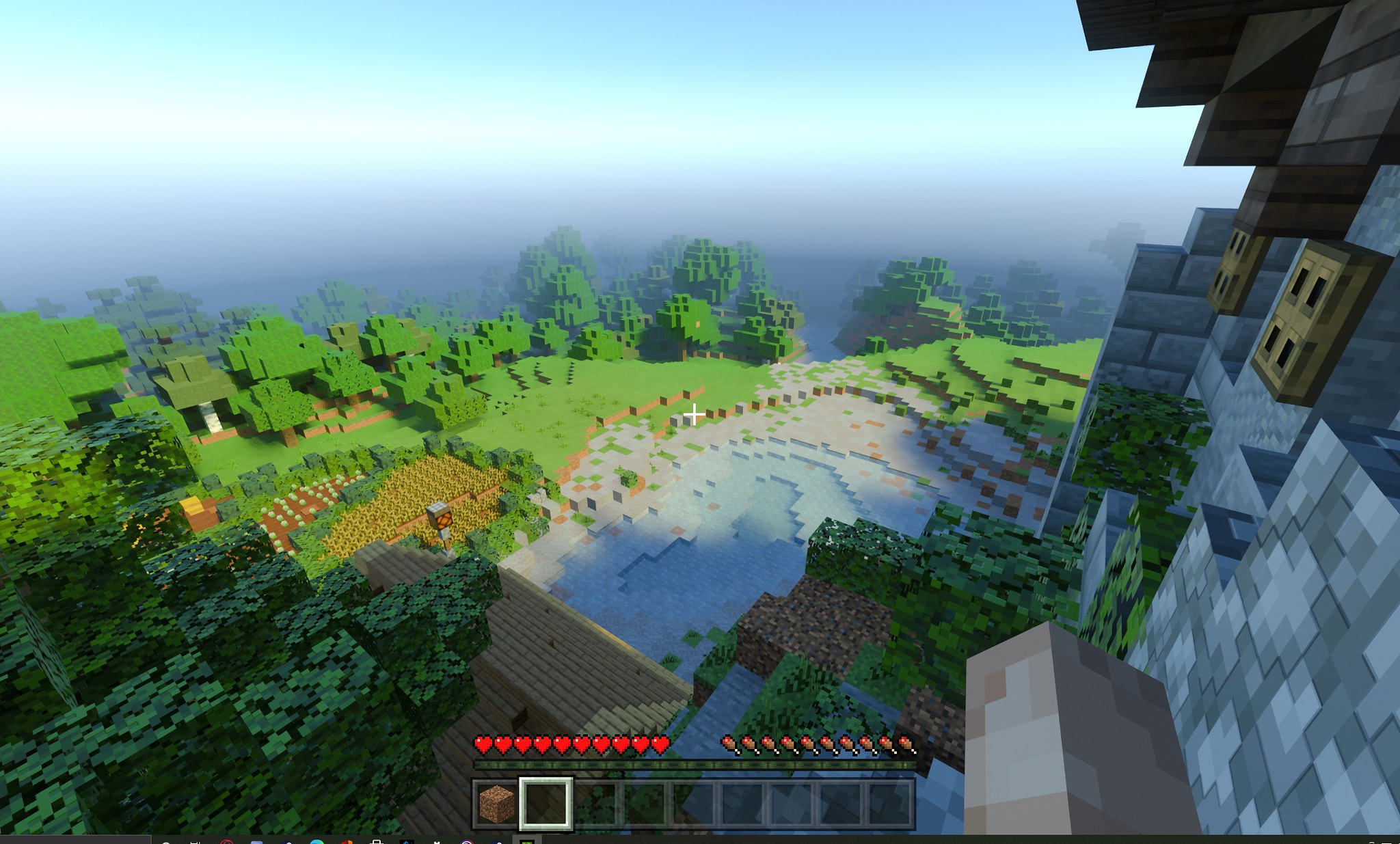This image captures an elevated view from a video game scene rendered in what appears to be a voxel or block-style, reminiscent of Minecraft. The sky, a gradient masterpiece, transitions from a lighter blue on the left to a deeper blue on the right, adding a sense of depth. Below, a stratified layering introduces a band of white transitioning seamlessly into a purplish-blue hue, enhancing the atmospheric dimension. 

The landscape presents a vivid mixture of blocky elements representing nature and structures. Dominating the lower part of the scene, a patchwork of small, cubic trees mimic a dense forest canopy. Scattered across are areas of lush green grass interspersed with darker green elements, potentially trees or bush-like formations, particularly noticeable in the bottom left corner, adding a touch of natural camouflage.

A shimmering pool is discernible amidst the foliage, bordered by a series of steps and more greenery, contributing to the scenic tranquility. Amongst this natural setting, stands a gray building topped with a brown, possibly thatched roof, situated towards the right-hand side of the image. The structure appears slightly weathered, with green moss or vine-like vegetation clinging to it, integrating the man-made with the natural environment seamlessly.